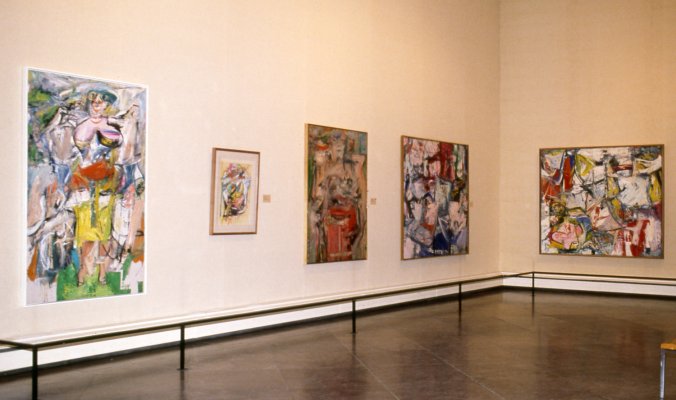The photograph showcases a corner of a museum gallery, featuring two tan walls with white trim at the bottom and a dark brown floor. The left wall displays four abstract paintings, while the right wall holds one. All the paintings, characterized by vague forms and vivid colors, seem to belong to the same artist due to their similar brushstrokes and style reminiscent of Picasso. One notable artwork on the left wall is smaller than the others but shares the same abstract subject matter. A sleek black rope fence, set low to the ground, cordons off the paintings, allowing a clear view while preventing visitors from getting too close. Predominant colors in the artwork include flesh tones, red, yellow, green, and brown, with the abstract compositions hinting at hidden shapes like a woman, a dog, and distant bushes.